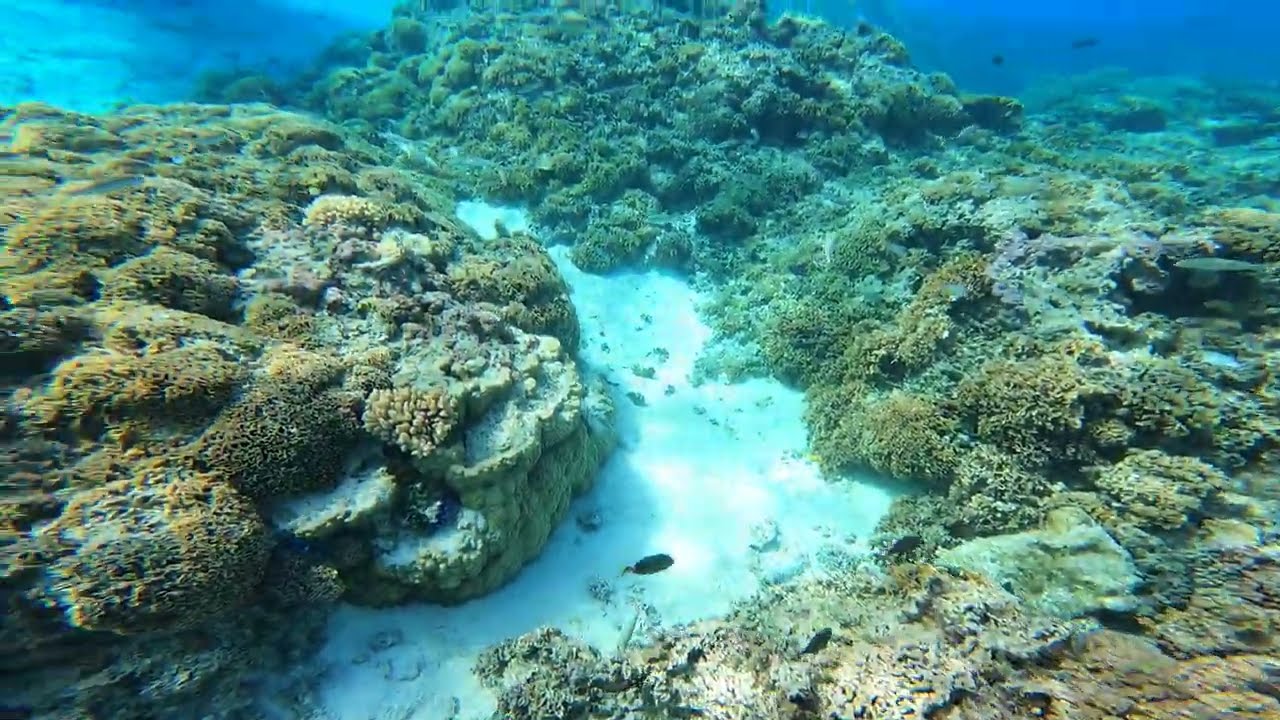The image is a horizontal rectangular underwater shot capturing the serene flow of a stream as it winds its way through moss-covered rocks towards a larger, calm body of water, presumably a lake. The aqua blue water is dotted with white spots and dark-colored fish, with the clarity suggesting a shallow depth of about 4-6 feet. The lake in the background, visible as the stream turns, reflects a darker blue hue with an unruffled surface, indicating a peaceful setting without waves. The underwater landscape is primarily composed of various shades of green moss, covering most of the rocks, with some bare rock patches and a few coral-like formations. The overall scene, bathed in natural light, emphasizes the vibrant colors and tranquil ambiance of the aquatic environment.